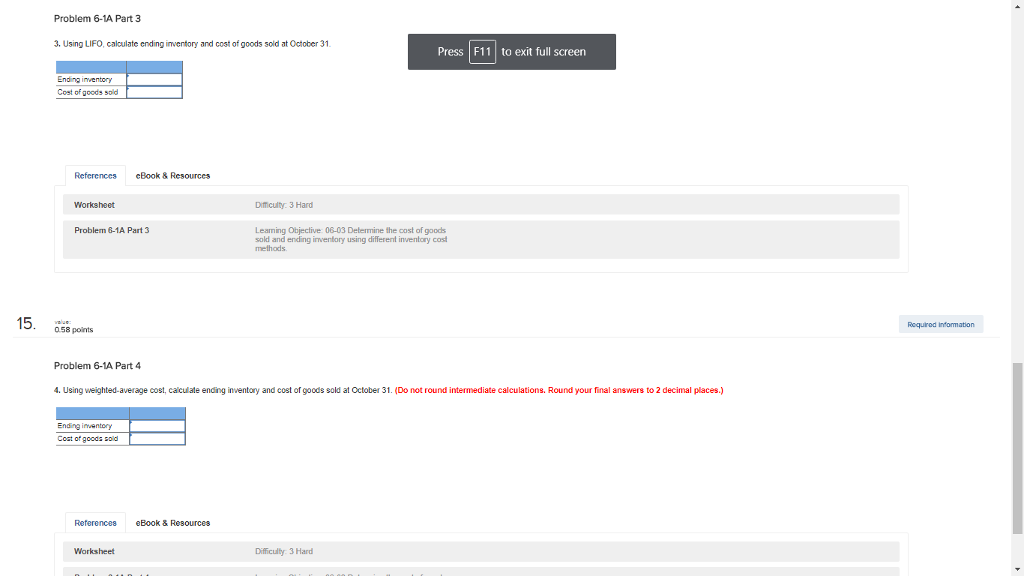A detailed caption for the described image could be:

---

This web page features a predominantly white background. In the top-left corner, bold black text titled "PROBLEM 6-1A" is prominently displayed, followed by "Part 3" in regular black font. Below this header, the text reads: "3. Using FIFO or LIFO. Calculate ending inventory and cost of goods sold at October 31st." 

Below this instruction, there is a small snippet of a spreadsheet, seemingly from Excel, showing two columns. The top of each column is dark blue. The first cell in the left column is labeled "Ending Inventory," and directly below it is "Cost of Goods Sold." The right column cells are currently blank. 

To the far right of the image, a black rectangle with white text indicates "Press F11" for full-screen mode (exit by pressing F11 again). This suggests the screenshot was taken on a desktop computer. 

Further down, a rectangle features alternating dark gray bands. The first, thinner band is about one-third the size of the second and contains bold black text that reads "Worksheet." To the right, in regular black text, it indicates "Difficulty: 3 (Hard)." 

The larger band below continues with "Problem 6-1A Part 3" in bold black, followed by a learning objective: "LO 606-03: Determine the cost of goods sold and the inventory using different inventory cost methods."

The top references section is noted as "Selected References" in blue text against a white background. Adjacent to this, there is a "15" in bold black, denoting "Value" and "0.58 points" also in bold black. 

Following this, "Problem 6-1A Part 4" appears, marked by the number "4" in regular black text. The task listed is: "Using weighted-average cost, calculate ending inventory and cost of goods sold at October 31st." Notably, instructions in red state: "Do not round intermediate calculations. Round your answers to two decimal places."

Lastly, the screenshot captures a section of a table, similar in format to the previous one, which is partially cut off. On the far right, a cyan blue rectangle labeled "Request Information" in dark blue text stands out.

---